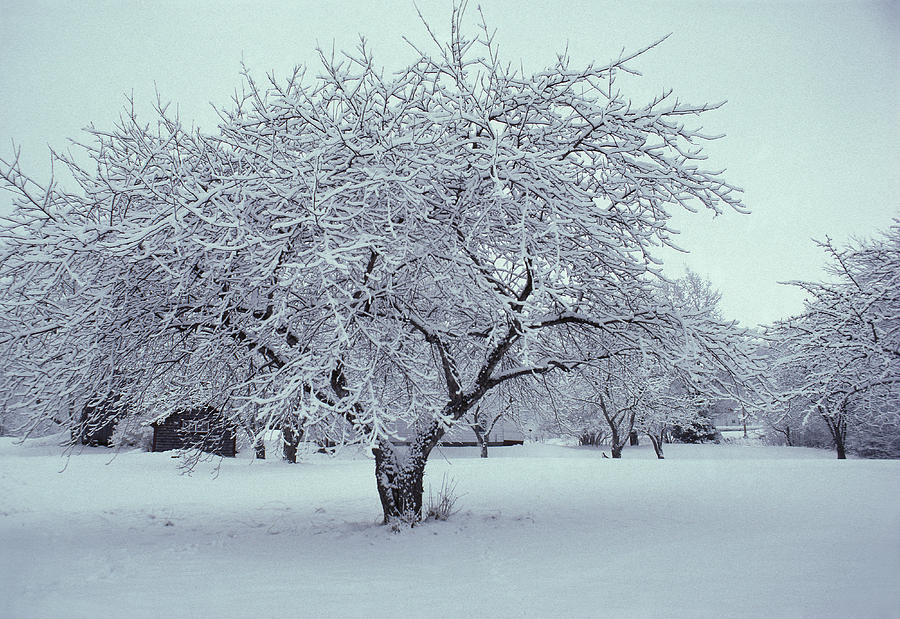This horizontally aligned rectangular photograph captures a serene winter landscape, possibly in a park or natural area. In the foreground stands the focal point, a relatively short tree with a thick, low trunk about four to five feet high, from which intricate branches extend outward and upward. These branches are bare, devoid of any leaves, and are heavily laden with snow and ice, creating delicate, frosty outlines. The ground below the tree is covered in a smooth, thick blanket of snow, with only a few subtle dents possibly indicating footprints right under the tree. The untouched snow forms small, gentle hills that recede into the background, which is filled with more evenly spaced trees, all similarly frosted and snow-covered. The sky above is a solid expanse of gray clouds, like a heavy blanket, adding to the sense of stillness and cold. Towards the back of the scene, a small brick structure, possibly a shed or cabin, stands quietly amidst the trees, with a fence and some other indistinct surroundings faintly visible further back. The overall scene is very tranquil and picturesque, embodying the calm beauty of a winter's day.